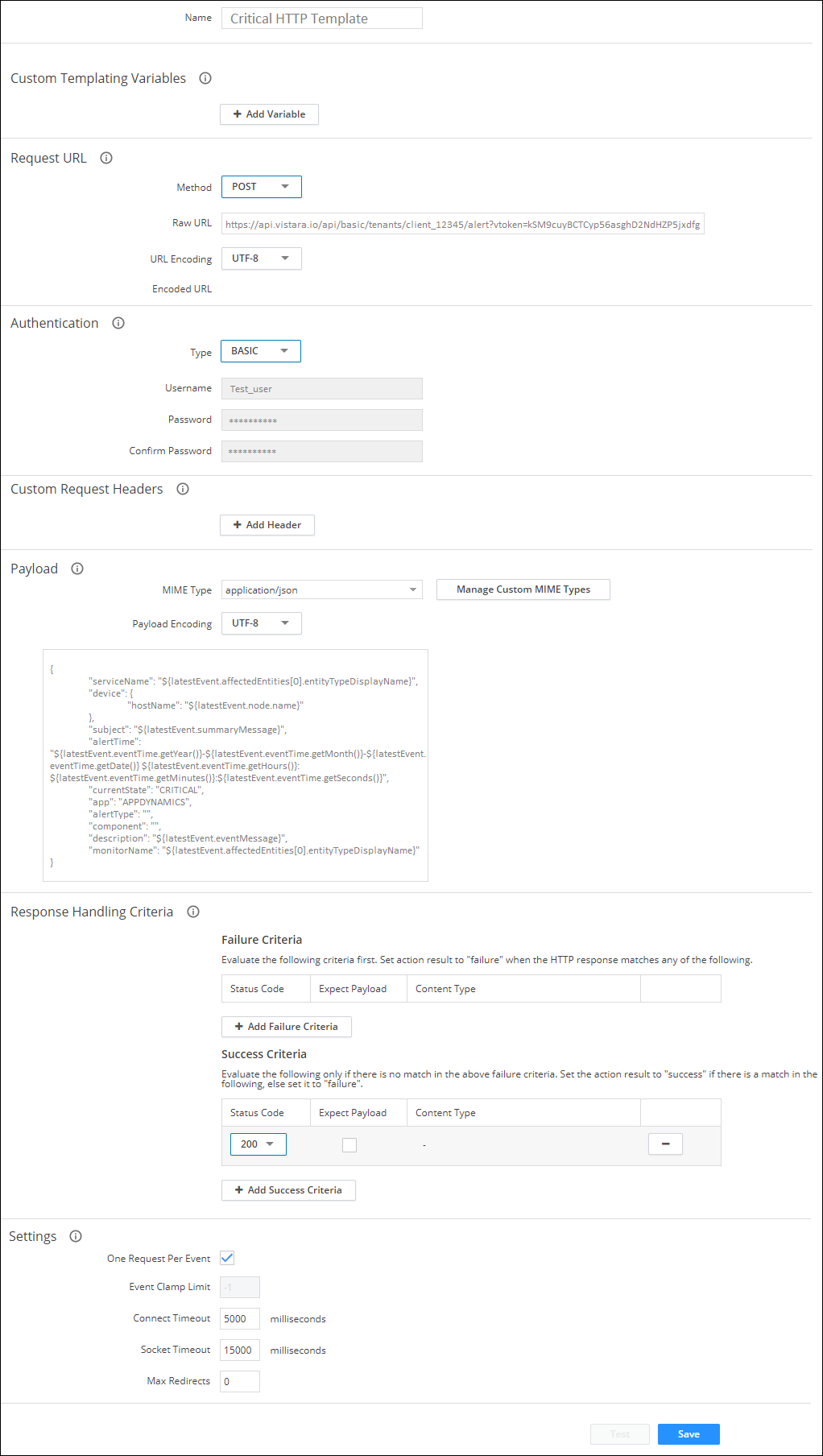The image displays a user interface on a white background, featuring several input fields and settings related to authentication and request configuration. 

At the top, there is a section for the Request URL and Authentication. Below that, there are fields labeled "Type," "Username," "Password," and "Confirm Password." Another area is designated for configuring custom request headers.

To the side, there is a box resembling a coding window, although the text inside is partly obscured. This box includes three words, the first starting with "R," the second with "H," and the third with "C." 

In the settings section, there's a gray rectangle with faint, unreadable text. Adjacent to this is a blue rectangle, prominently featuring the word "Train" in white text.